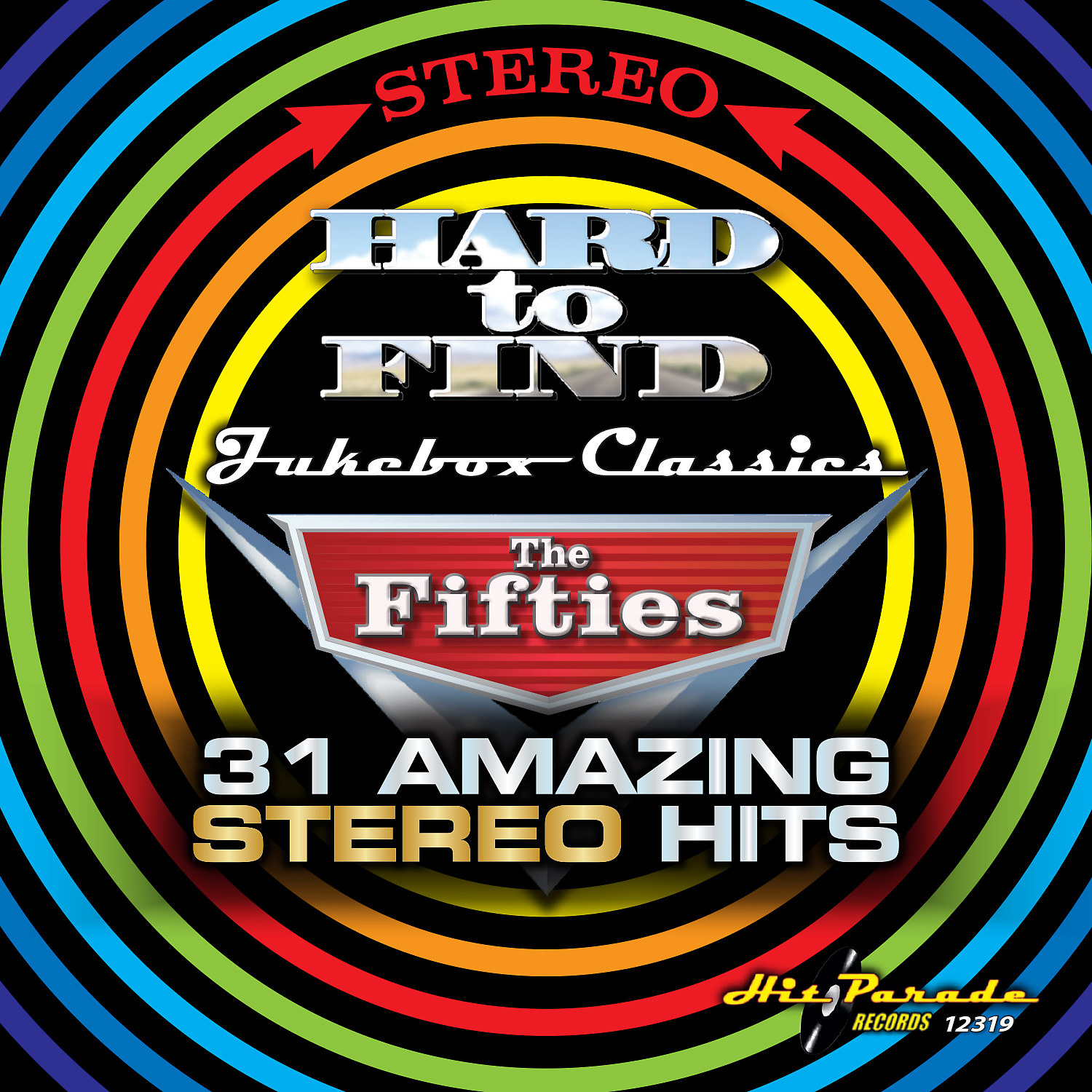The image, which resembles a digitally created poster, features a background that is completely black. In the foreground, a series of concentric circles radiate outward from the center, transitioning through vibrant colors from yellow, orange, red, green, light blue, dark blue, to purple. In the very middle of the image, within the red circle, bold red text reads "STEREO." Directly beneath this, in a shiny chrome-style font, stands the phrase "HARD TO FIND." Below it, "JUKEBOX CLASSICS" is displayed in a stylized, script-like font reminiscent of the 1950s. Further down, centered on a red, trapezoidal background with silver borders, the text "THE 50s" is written in silver, followed by "31 AMAZING STEREO HITS" in white text, with "STEREO" highlighted in gold. In the lower right-hand corner, a small logo in yellow text reads "Hit Parade Records," accompanied by the number "1 2 3 1 9" in white text, and features a small image of a record between the words "Hit" and "Parade."